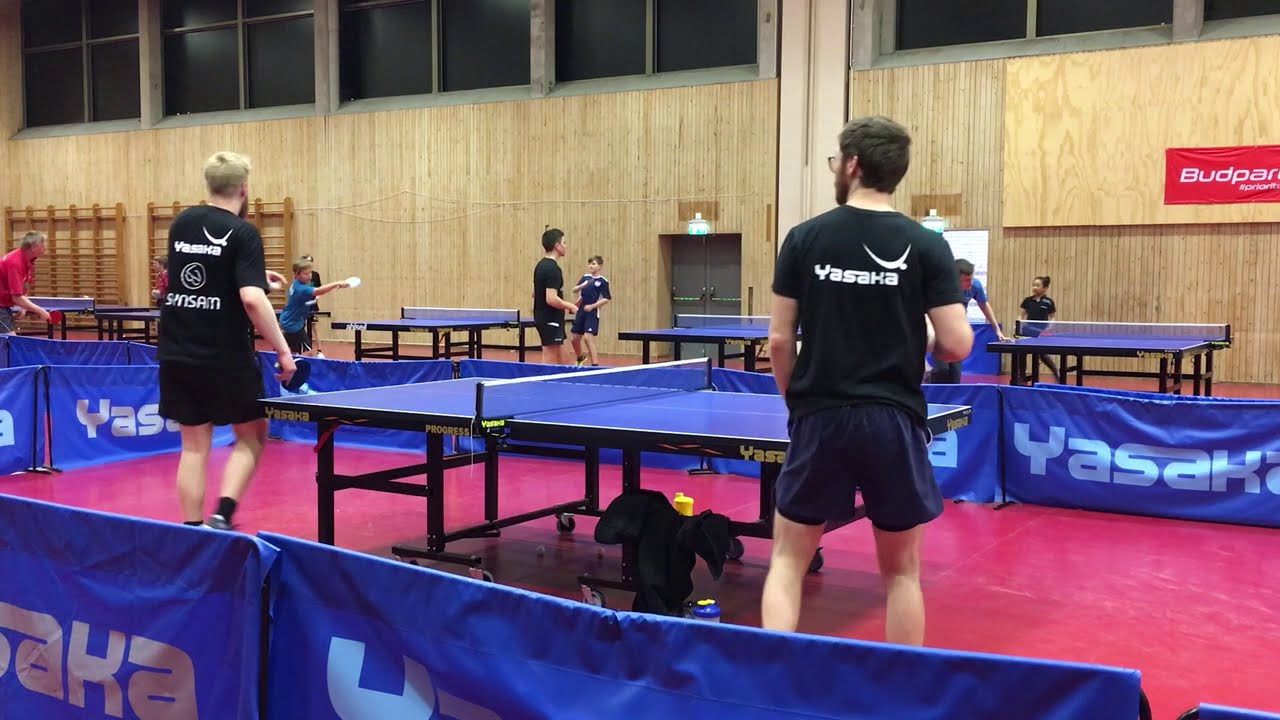The image captures an indoor ping-pong tournament set in a gymnasium with a prominent wooden wall and large windows. At the forefront, two men in their late twenties or early thirties are engaged in a game, both wearing black Yasaka shirts and blue shorts. The central ping-pong table they are playing on features a blue surface with a white net and a black base, surrounded by a hip-high blue divider. Behind them, a series of four additional tables are occupied by players of varying ages and skill levels, including two young boys about ten years old. The gymnasium floor is a striking red, contrasting with the light brown wood slats of the wall and the gray window frames above. A partially visible banner on the wall reads "Budpa" and "Kadaw." The setting is dynamic, with players in black, blue, and red shirts, emphasizing the competitive atmosphere of the tournament.